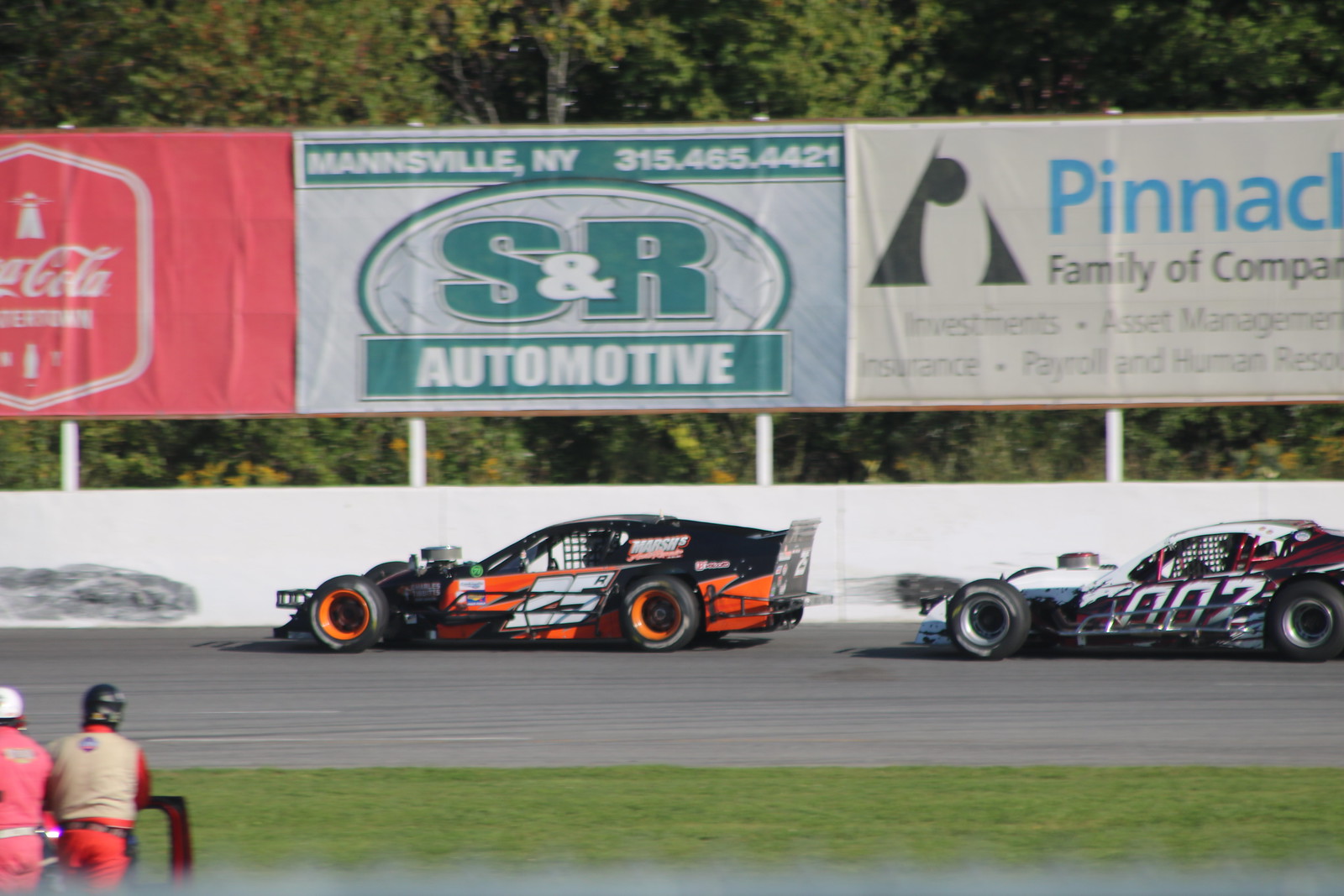This horizontally oriented photograph captures an exciting race scene on a gray track flanked by a stretch of green grass in the foreground. Two race cars are speeding down the track; the lead car is black and orange with the number 25 prominently displayed on its side, while the car trailing behind is primarily white and black, featuring the number 007 on its side. In the bottom left corner of the image, two gentlemen, perhaps pit crew or spectators, stand facing away from the camera. Above the track, three large billboards dominate the top of the photograph. The first billboard, on the left, advertises Coca-Cola with white text and a bottle image. The middle billboard reads "S&R Automotive" in green and white text, and the right billboard, characterized by a triangular logo, promotes "Pinnacle Family of Companies." Lush green foliage from nearby trees frames the scene, suggesting it is a vibrant summer day.